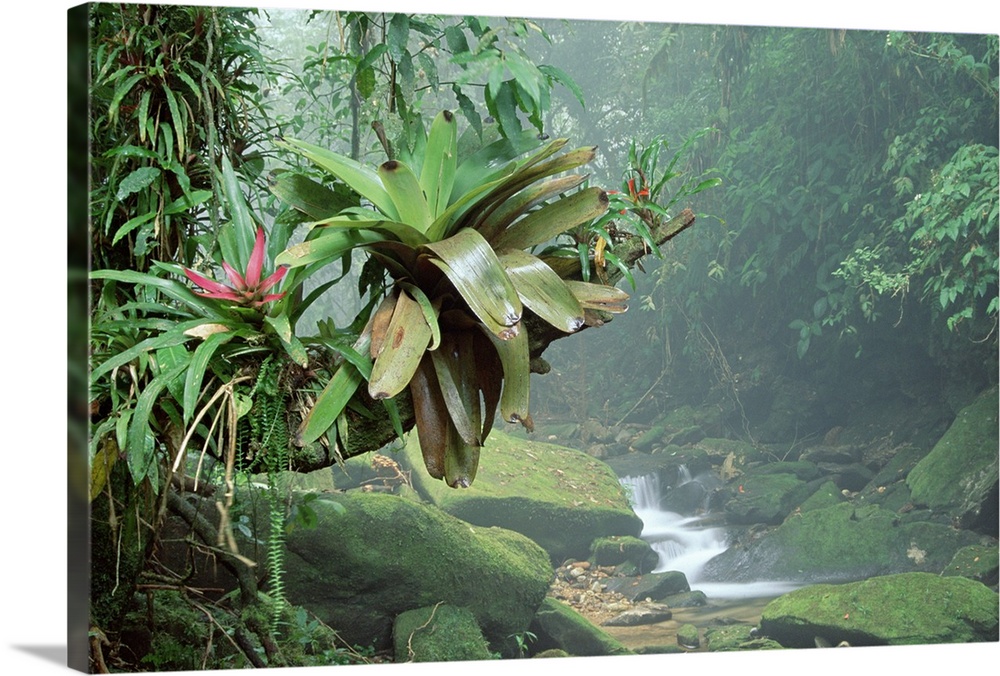The image is a stunning, tranquil depiction of a tropical landscape. Dominating the scene is a cascading waterfall that flows into a mist-covered stream or river, creating a peaceful atmosphere. Surrounding the waterfall and water are lush green trees and foliage, including a tree trunk on the left adorned with various plants, some with vibrant red flowers. Moss-covered rocks line the stream, adding to the natural beauty of the scene. On the left side of the image, a large, curvaceous branch extends into the center, covered in massive, fan-like banana leaves, some verdantly green while others show signs of browning. Vines and fern-like plants drape gracefully around the branch. Additionally, a cluster of pink flowers and ferns can be seen on the left, further enhancing the idyllic setting. The entire composition is reminiscent of a wrapped canvas artwork, capturing the essence of Mother Nature in its serene, picturesque splendor.